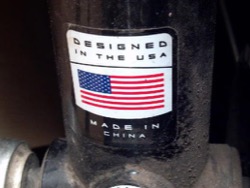The close-up image showcases a cylindrical vacuum cleaner, covered in both light and dark brown dust, giving it a weathered and dirty appearance. The vacuum has a distinct protruding cylindrical pipe, black in color but blanketed in light brown dust, leading to a slightly rusted and chipped light blue section. Above this, there is a prominent clear cylindrical component adorned with a noticeable sticker. The sticker features a design with a large black rectangle containing a smaller white rectangle inside. Within the inner rectangle, the text reads "DESIGNED IN THE USA" in black capital letters. Beneath this, there is a black dividing line followed by a depiction of the American flag—a dark blue rectangle filled with white dots symbolizing stars on the left, and red and white stripes extending horizontally. Below this, the words "MADE IN CHINA" are inscribed in white capital letters on the black background. The vacuum and its sticker give off an impression of a well-used yet internationally crafted appliance.